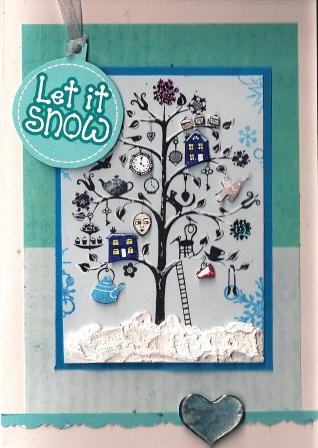The image depicted is a whimsical greeting card set against a white background. The greeting card has a vertical rectangle layout, with a notable feature being a circular tag at the top left corner that reads "Let it Snow" in white text. This tag is blue and attached with a ribbon. The card is divided visually, with the top half shaded in darker green and the bottom in a light white-blue tone. 

In the central portion of the card, there is a smaller, vertically-oriented rectangle outlined in blue, featuring a black tree with multiple branches. The tree is adorned with various hanging objects such as a pale mannequin face, a blue teapot, a golden trumpet, a black house, and a white clock, symbolizing the effort put into decorating it. At the base of the tree, there is a black ladder and scattered white snow. Additionally, a blue ribbon strip runs along the very bottom of the card, culminating in a glossy blue heart positioned at the bottom right corner.